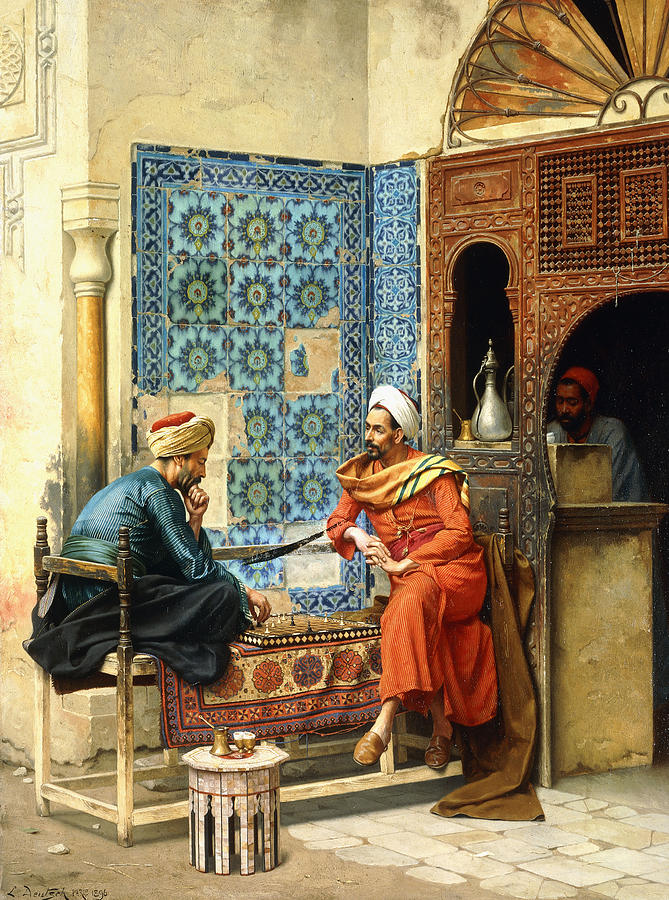The painting depicts a historical Middle Eastern scene where two men are engrossed in a game of chess on a bench outside a building. The man on the left is wearing a blue robe and a turban, sits cross-legged, while the man on the right, dressed in an orange robe and turban, sits with his legs crossed. Both men are deeply focused on the chessboard, which is placed on a vibrant rug beneath them. Nearby, a small table holds a few items, including two gold cups and a larger gold container. The backdrop features a cream-colored wall adorned with blue tiles behind the bench, and some brownish-red decorative tiles at the front. Through the building’s gate, a worker, dressed in blue with an orange hat, stands at a counter next to a silver kettle, appearing as if he might be serving drinks. The artist's name is inscribed in the bottom left corner of the painting.